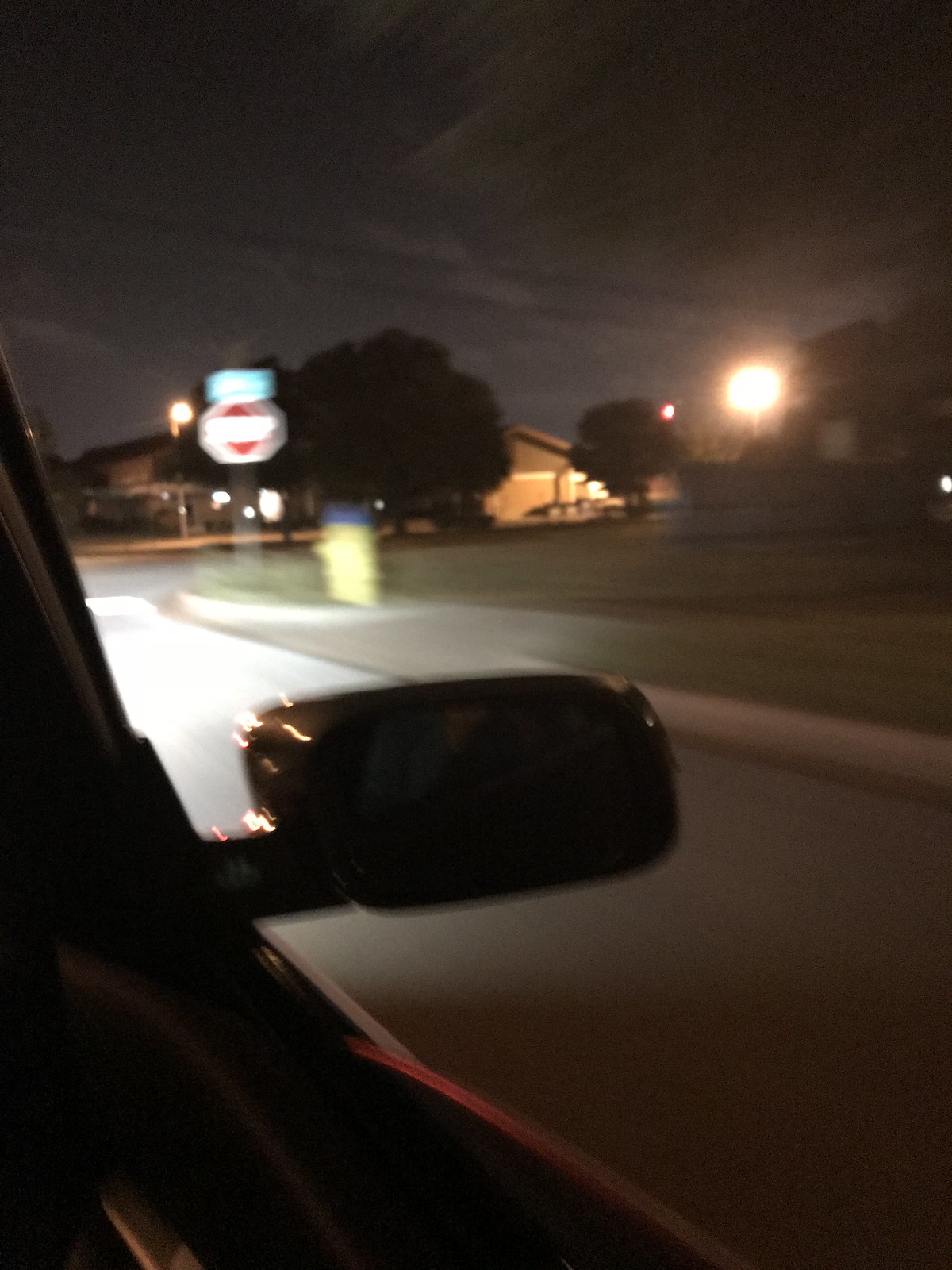Captured from the passenger's window, this nighttime image portrays the view just before reaching an intersection. The car's rearview mirror and the frame of the window are in sight, framing a tranquil residential neighborhood. A stop sign, crowned with a street name sign, stands prominently at the corner. Near the sidewalk, a yellow fire hydrant glows faintly under the streetlights. Ahead, single-story homes with trees adorning their lawns punctuate the scene. To the immediate right, a flat field stretches out, fronted by a sign that suggests it might be a school. The dark sky is softly illuminated by the street lamps, enhancing the serene, peaceful atmosphere.